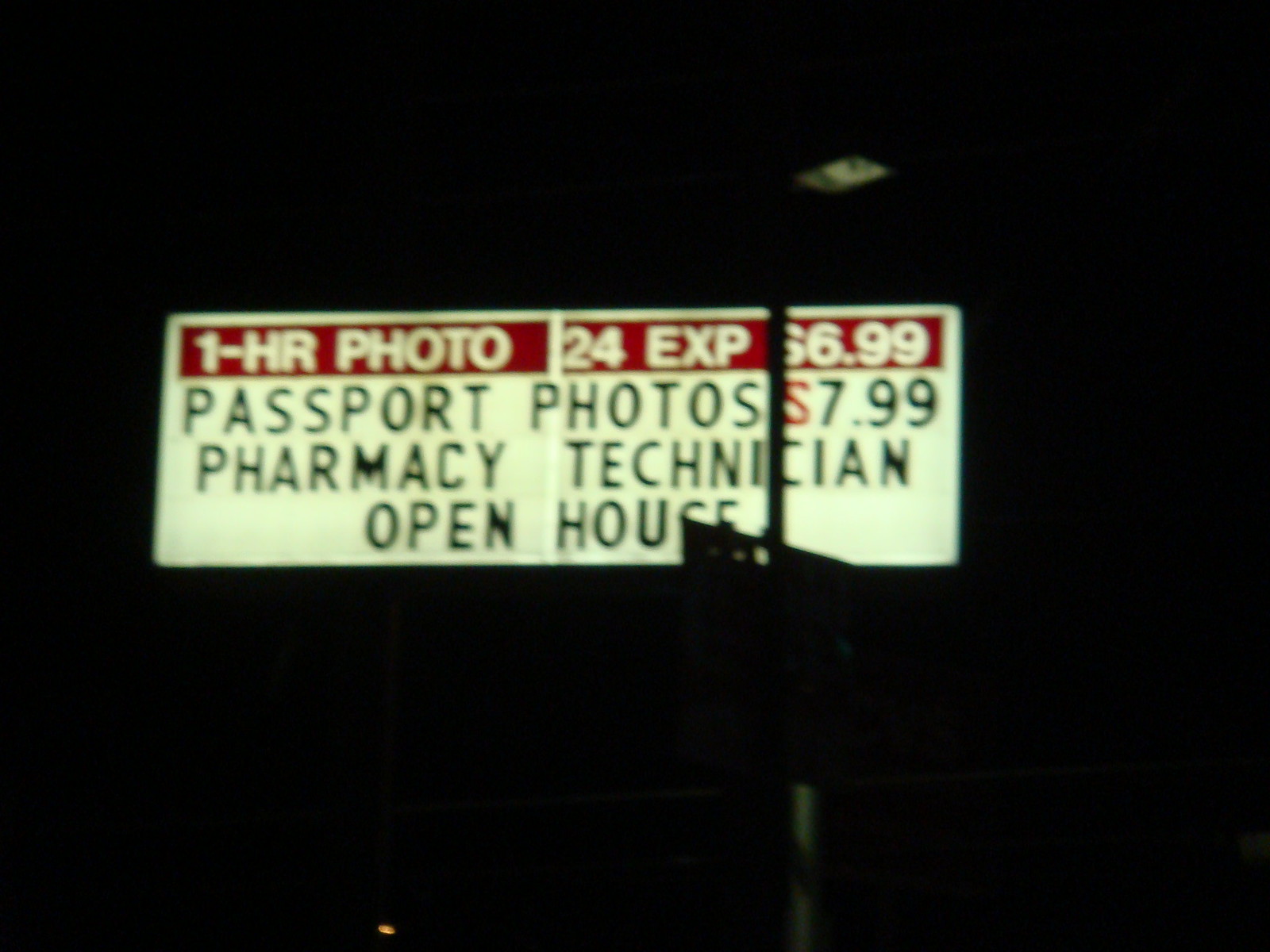This image, though blurry and low in resolution, features a rectangular, lit-up billboard centered within a dark, square frame. The billboard's upper section sports a deep red background, with the text "1-HR Photo 24 EXP $6.99" boldly displayed in white. Below, a contrasting white section showcases three lines of black text that advertise "Passport Photos $7.99" and "Pharmacy Technician Open House," with the dollar sign rendered in an eye-catching red hue. Despite the fuzziness and low-quality nature of the image, the illuminated billboard stands out clearly, offering a glimpse into its promotional content.